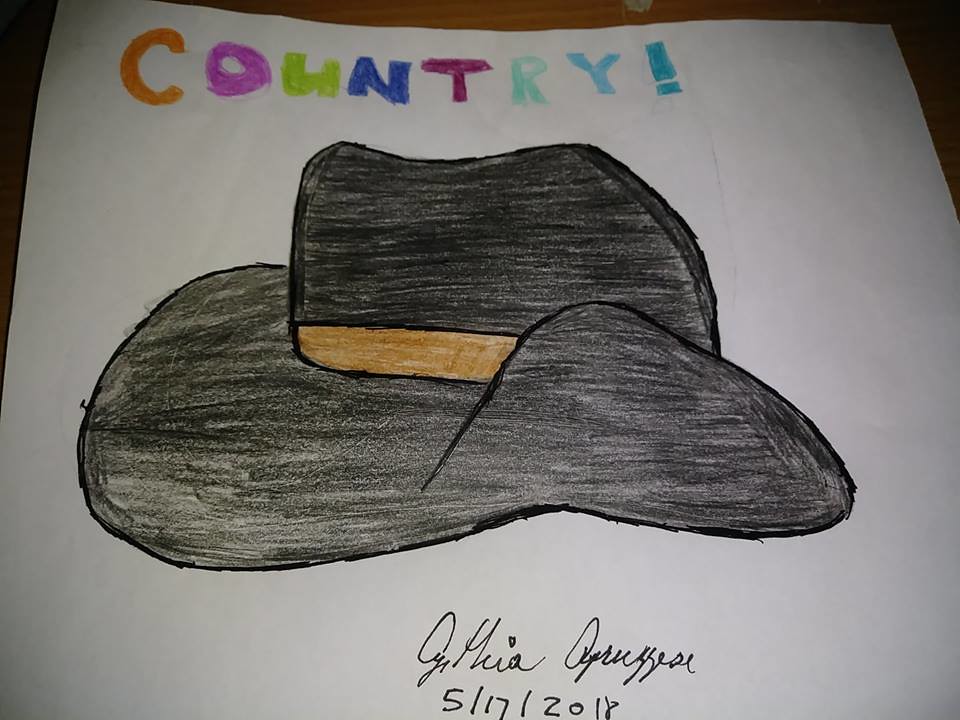Photograph of a colored pencil drawing on a white sheet of paper, resting on a brown table with a narrow border visible along the top and sides of the frame. The drawing, likely created by an older child, features a black cowboy hat with a golden band. The hat's brim is folded upward, especially pronounced on the left side. Above the hat, the word "COUNTRY" is written in vibrant, multicolored letters: orange, pink, lime green, royal blue, maroon, mint green, light blue, and a teal exclamation point. The bottom of the drawing is signed in cursive by "Cynthia," though the last name is illegible, and dated 5-17-2018.